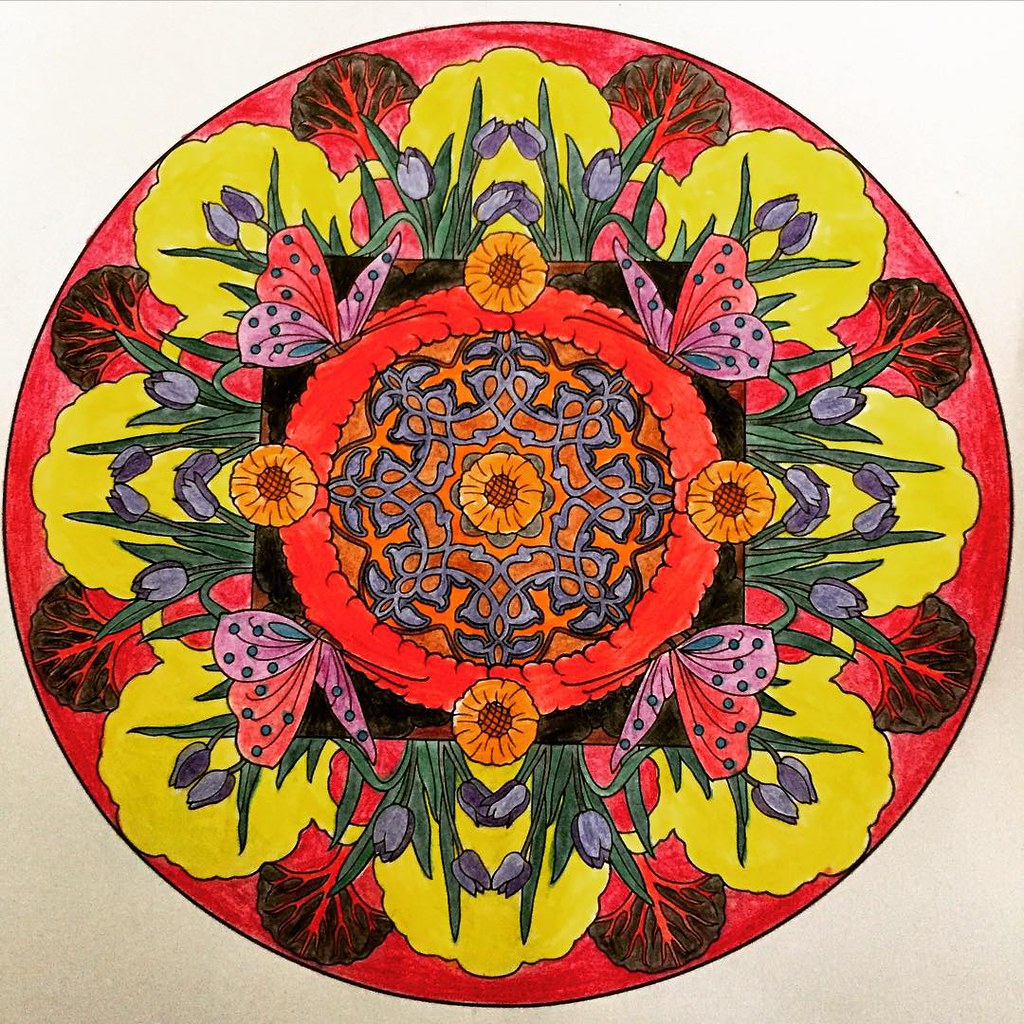The artwork features an intricate and vivid composition. The edges of the piece are adorned with white and brown hues. Moving inward, a prominent red circle dominates the central area. Surrounding this circle are clusters of multiple flowers, interspersed with illustrated trees, each depicted with branches and black leaves. Additionally, bright yellow puffs radiate around the center, complemented by green leaves and purple blossoms.

In the vicinity of the center, a black square is noticeable. Around this square, particularly on the top left, a vibrant red ring encircles the area, with sunflowers positioned at the cardinal points—north, south, east, and west.

The upper left corner showcases a beautifully detailed butterfly with purple wings accented by red and blue dots, and a brown body. The upper right mirrors this butterfly design, also with a brown body, purple wings, and blue dot embellishments. The lower left corner introduces another variation with pink, blue, and red colors.

At the core of this composition, there's a distinct pattern that culminates in the very center with a radiant sunflower, characterized by its yellow petals and a deep brown center, serving as an eye-catching focal point.